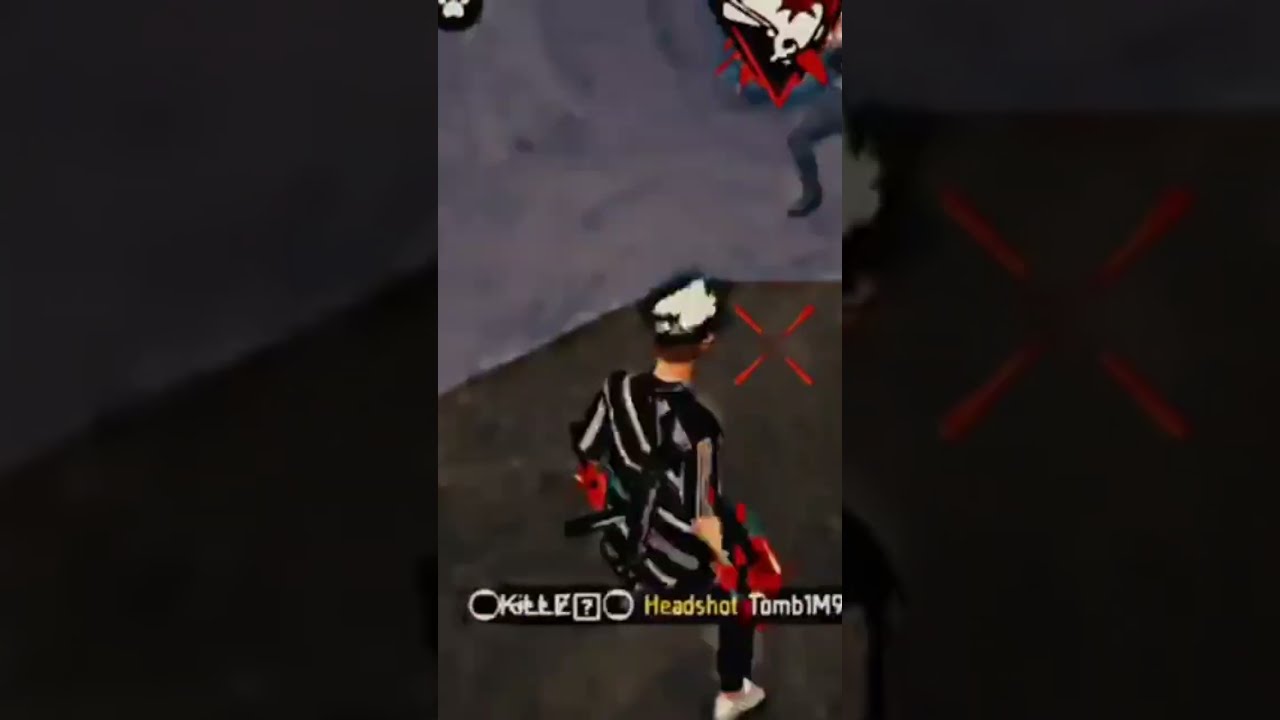In this video game screenshot, we observe a bird's-eye view centered on two characters standing on a gray pavement that transitions from dark gray at the bottom to lighter gray at the top. The primary character, closer to the viewer, is adorned in a black and white striped shirt, white shoes, and a black hat with a white pattern. Notably, this character also has brown hair, fair skin, and a gun, possibly a submachine gun, strapped to their back. Hovering over this individual at the bottom of the image is a banner partially obscured by symbols and letters, containing the words "HEADSHOT" and "TOMB 1M9" in a combination of white and yellow text. 

Nearby, a red four-pointed star or cross is marked on the ground next to the character's head, indicating a point of interest or interaction. In the distance, another character is partially visible, showing only a leg and what appears to be a shield, and possibly wearing a white animal mask. The left and right borders of the image feature enlarged, darkened, and less defined versions of the primary scene, emphasizing the significant elements like the ground color transition and the red cross.

The overall style of the image is reminiscent of a video game illustration, with its detailed character design and text elements suggesting an action or combat scenario within the game environment.